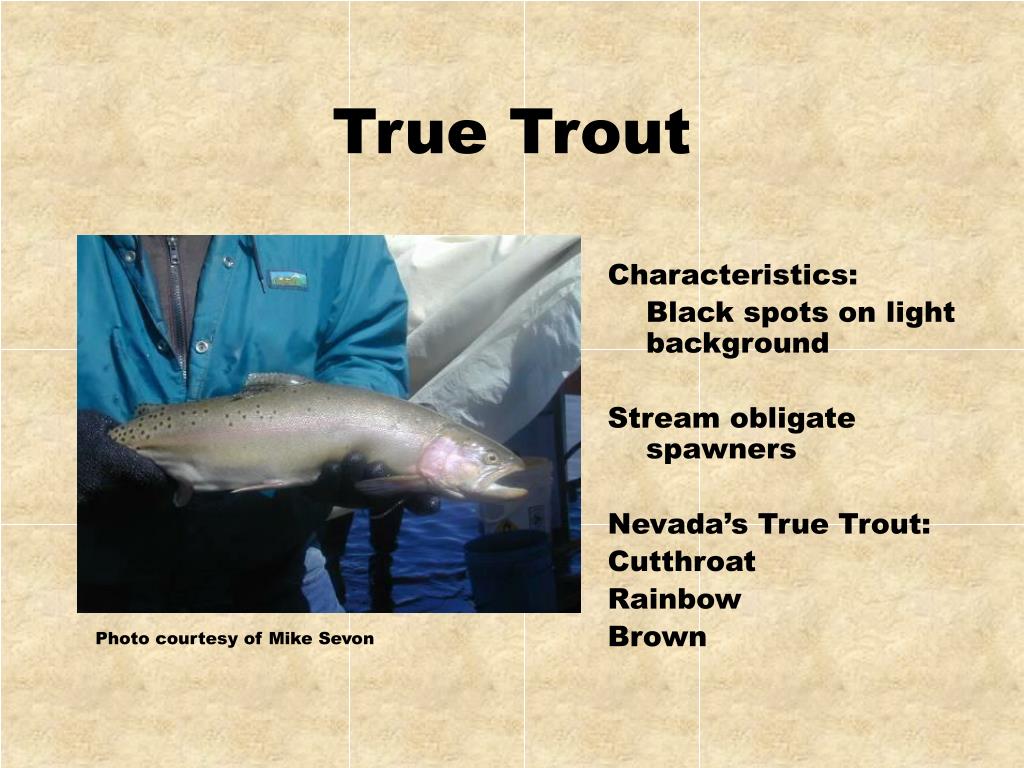The image features a beige background with a centrally placed, prominent title in large font reading "True Trout." On the left side, there is a photograph of a man, who is partially shown, wearing a white or teal jacket and black gloves, holding a silver trout fish. The man's face isn't visible, but the fish is clearly depicted, with its mouth open and head pointing to the right. The backdrop of the photograph includes water, indicating the man is likely on a boat, engaged in fishing. Below the photograph is a photo credit: "Photo courtesy of Mike Savon.”

To the right of the photograph, there are three paragraphs of text: 
1. "Characteristic black spots on light background."
2. "Stream obligate spawners."
3. "Nevada's true trout: cutthroat, rainbow, brown."

The scene is set outdoors, in a fishing context, with the detailed information about the different types of trout provided alongside the image. The colors present in the image include tan, black, blue, gray, silver, and white.